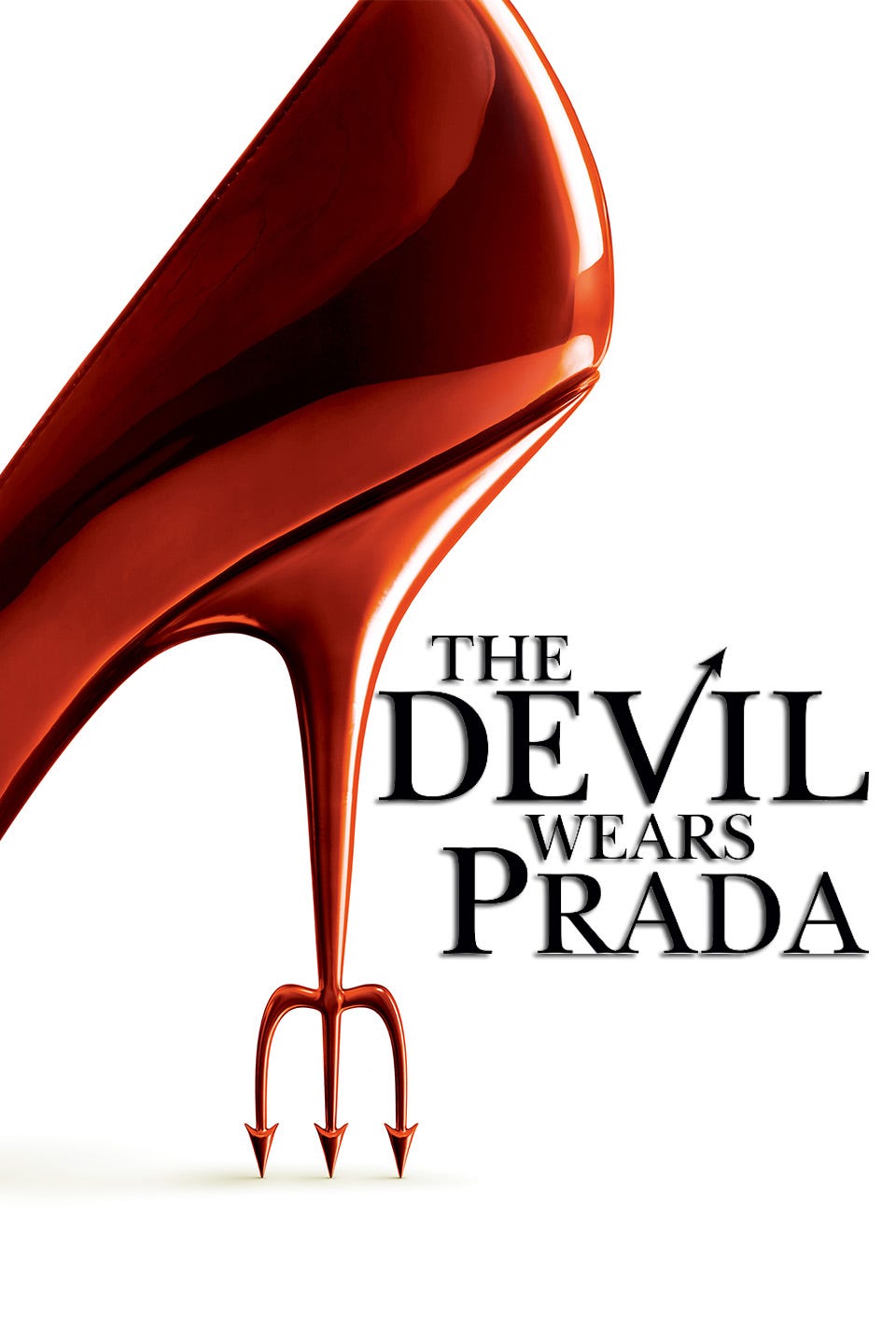The poster advertises the movie "The Devil Wears Prada" and features a sleek, minimalist design set against a pure white background. On the far left, a glossy red high heel dominates the image, its heel cleverly transformed into a menacing, three-pronged devil's pitchfork. To the right, the movie title is prominently displayed in large black letters. The text arrangement emphasizes key words: "The Devil" in large font, with the "V" in "Devil" modified to resemble an arrow or a devil's tail. Below "Devil," the smaller word "wears" leads to the final large, bold word "Prada." The simple yet striking composition effectively highlights the movie's title and the devilish theme, using a minimalistic but powerful visual style.